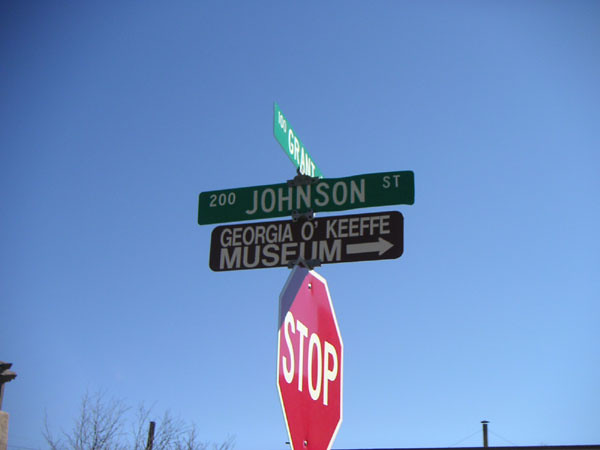In this vibrant photograph, a picturesque blue sky serves as the backdrop. The upper edges of the frame are adorned with the tops of lush green trees, conveying a sense of tranquility and natural beauty. To the right, the corner of a house subtly peeks into view, adding a touch of domestic charm to the scene. Stretching across the sky are a couple of power lines, introducing an element of urban life.

Dominating the lower part of the image is a prominent red stop sign with a white border, featuring bold white letters that command 'STOP.' Attached to the stop sign pole are three green street signs with white text. The middle sign directs visitors to the Georgia O’Keeffe Museum, indicating a right turn. Above it, another sign denotes '200 Johnson Street.' The topmost sign, oriented in the opposite direction, reads 'Grant Street,' providing clear navigation details. This convergence of nature, urban infrastructure, and directional signage creates a dynamic and informative snapshot of a specific locale.